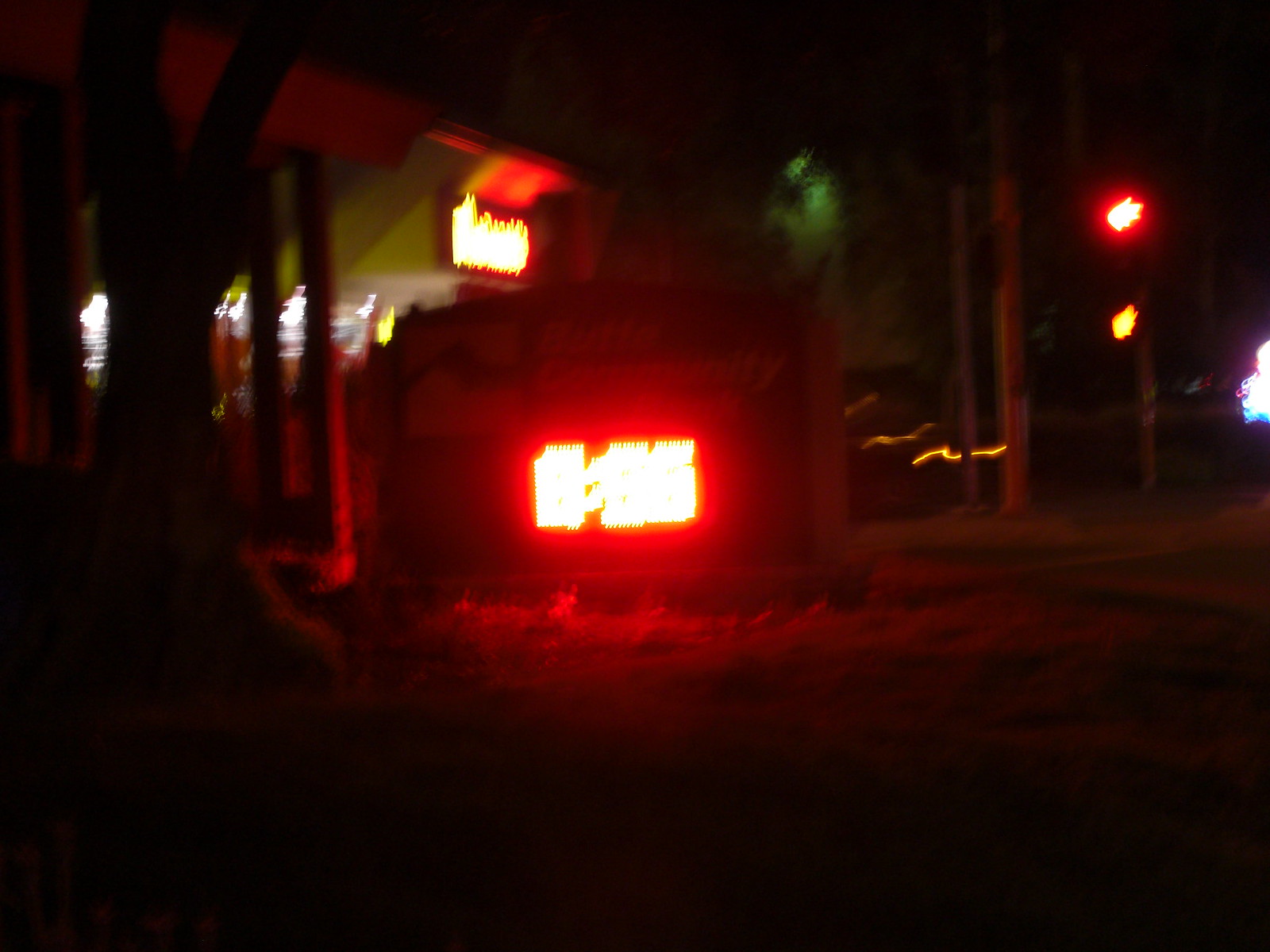In this blurry nighttime street photo, the focal point is a sign with partially legible text including the word "community." The sign is illuminated by a bright reddish-orange glow in the center and additional red lights at the top left and right corners. The scene is predominantly dark, with details difficult to discern. Underneath the sign, there is a patch of dry grass scattered on the ground. To the left and right of the sign are poles, with a turn signal or walk signal lamp visible near the right edge. A tree stump is faintly visible on the left, and a green tree is present in the background. A building with a neon sign is also situated behind the main sign. The overall composition creates a moody atmosphere due to the obscured visibility and dark backdrop.